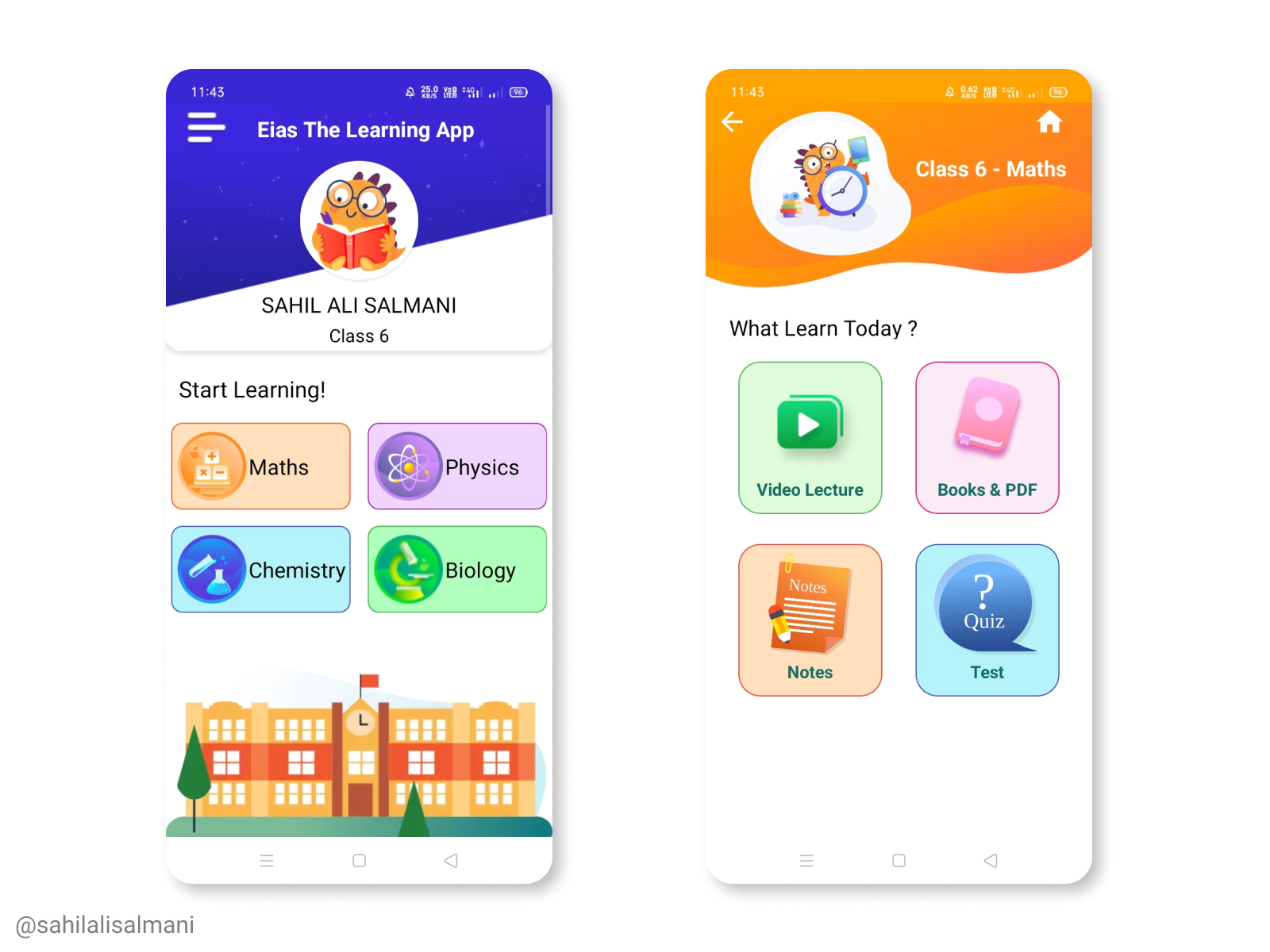The side-by-side images appear to be screenshots from an educational application called EIAS (E-I-A-S), known as "the learning app." The first image features a brightly colored, cartoonish interface with the app's title prominently displayed. Below the title, there's an adorable cartoon avatar of a reading dinosaur wearing glasses and holding a book. The avatar is labeled with the name "Sahil Ali Salami, Class 6."

Beneath the avatar, there are four vibrant options under the heading "Start Learning!" Each option is color-coded and represents a different subject: 
1. Maths
2. Physics
3. Chemistry
4. Biology

Additionally, a charming cartoon image of a school, surrounded by trees, is visible at the bottom of this first screen.

The second image, positioned directly next to the first, also belongs to the EIAS app. It is focused on the "Class 6 Maths" section. Under the heading "What Learn Today?" four colorful learning options are offered:
1. Video Lecture (green)
2. Books and PDF (pink)
3. Notes (pink and orange)
4. Test (featuring a speech bubble with a question mark labeled "quiz")

These screenshots collectively highlight the app's engaging and educational interface designed to encourage learning for Class 6 students.